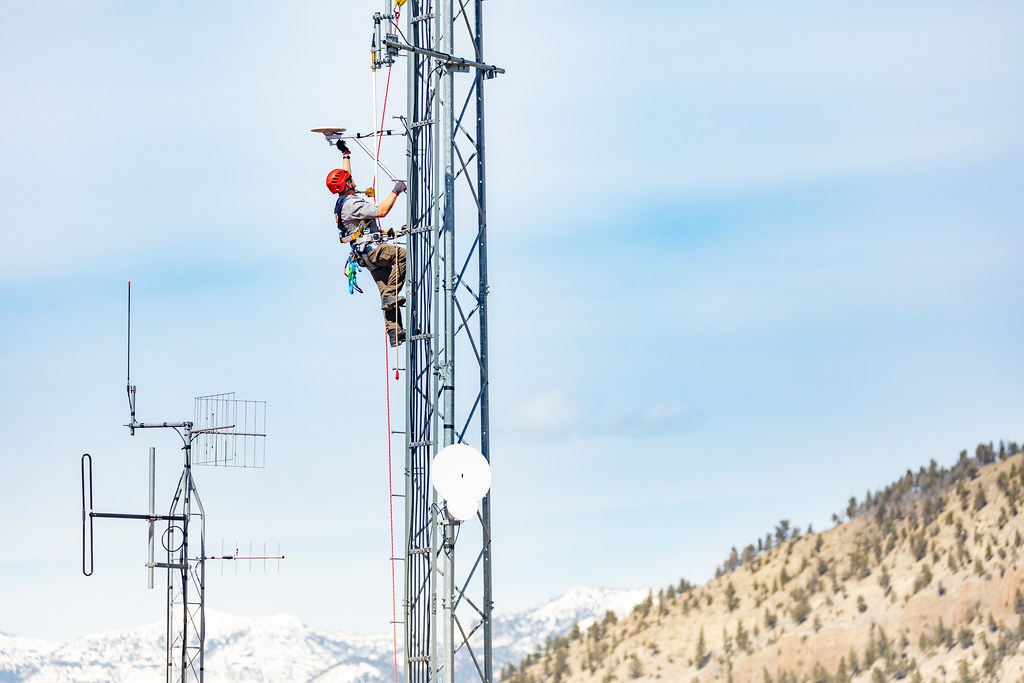In this striking photo, a technician is seen scaling a tall metal cell phone tower, harnessed securely for safety. Clad in a red helmet, a gray shirt, and tan pants, he diligently works high above the ground, with red and white safety cables ensuring his protection. His hands grip a device, possibly a tool essential for his task. The backdrop features a breathtaking landscape with a bright blue sky that dominates the majority of the background, punctuated by a few clouds in the lower left corner. To the right of the towering structure, a dusty, tree-covered mountain stands prominently, while snow-capped peaks can be seen in the distance, adding an element of dramatic contrast to the scene. Additionally, another smaller metal tower is situated to the left of the technician, highlighting the expanse and complexity of the technology he is maintaining. The visual perspective emphasizes the significant height at which he is working, parallel to the adjacent mountain range.